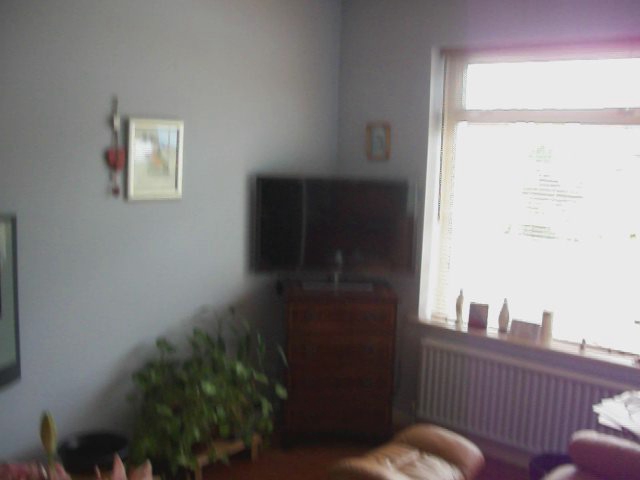In this image, a living room is prominently featured, centered around a small LCD TV positioned in the corner atop a dark cherry orchard dresser with four drawers. To the right of the TV, an open window with blinds halfway drawn allows light to stream in, illuminating several small figurines and bottles on the windowsill. Below the window, a heater with visible vents is mounted to the wall. On the bottom right, a cross-sectional view of a brown leather recliner with a separate footrest is visible. To the left of the TV, a fake green potted plant rests on a small wooden stool on the floor, and above it hangs a blurred picture frame on the wall. The overall scene provides a cozy, lived-in atmosphere despite the slight blurriness of the image.